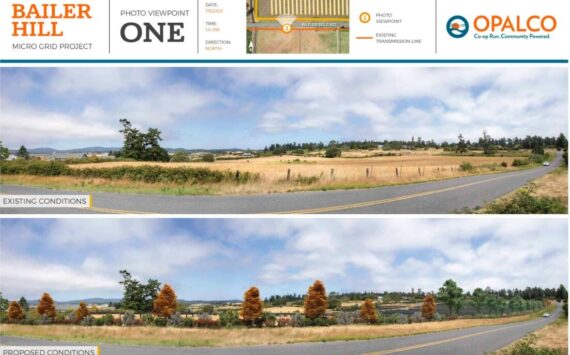This advertisement highlights the "Baylor Hill Microgrid Project," with emphasis on Photo Viewpoint 1. The display contrasts two images: the "existing conditions" at the top and the "proposed conditions" below. Both images capture a curved road flanked by a brown grassy field with a car approaching. Behind the roadside in the top image, sparse trees frame the landscape against a blue sky. In the bottom image, which details the "proposed conditions," there is a noticeable increase in greenery with more trees lining the roadway. The advertisement features labels and text including "Opalco Co-op Run Community Powered," accentuating the project's commitment to enhancing the landscape through new developments.